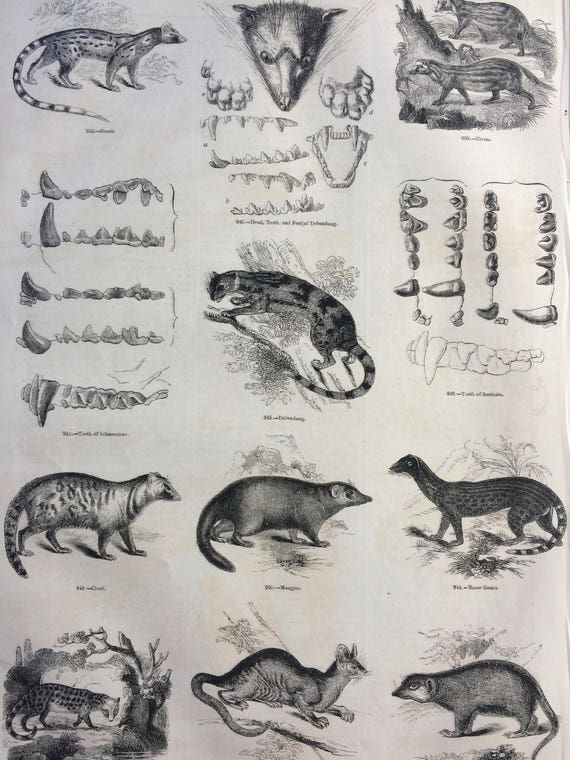This black-and-white illustration resembles an old-time educational poster, featuring a detailed diagram of different weasel-like and cat-like animals arranged in a grid of three columns and four rows. The entire image is intricately drawn, suggesting it is an older piece, with minimal white space between the drawings.

In the top row, three weasel-like animals are depicted, with the one in the center shown face-on, complete with a detailed view of its teeth and paws, and the ones on either side facing left. The second row includes detailed drawings of teeth—with particular emphasis on pointy canines—and in the center, another cat-like creature with stripes. The right side of this row also shows another detailed illustration of teeth.

Below this, in the third row, there are three more illustrations of the weasel-like animals with varied postures, including one perched on a tree branch. The bottom row features another set of these animals in different positions. Two animals on the top right corner are turned to the left, and an animal is seen prominently on the bottom right, viewed from the side.

Despite the intricacy, the writing on the image is not legible, lending a mysterious and aged quality to this ornate diagram.